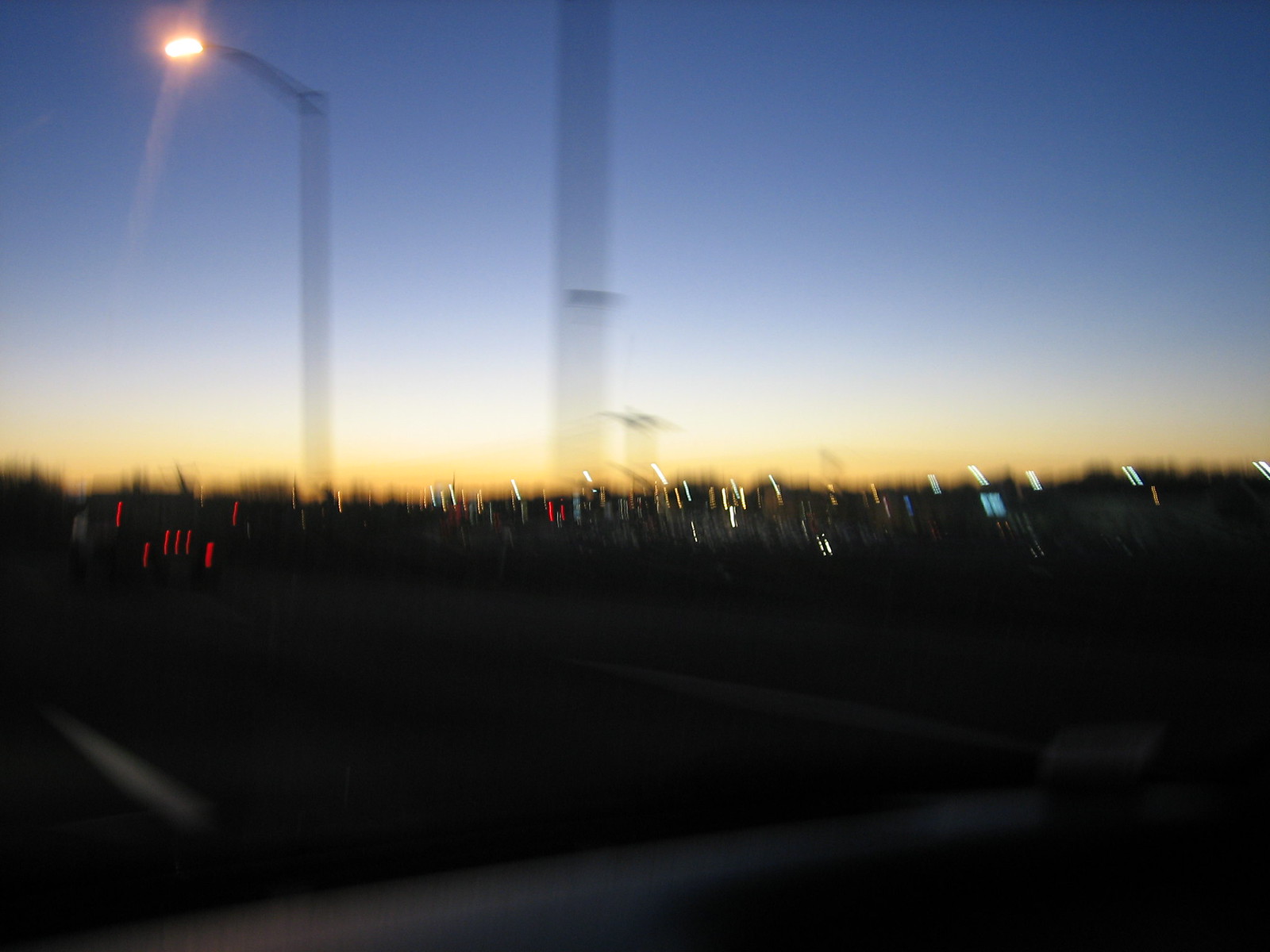This square-shaped image, though blurry and of low resolution, captures an outdoor scene. The top half of the picture is dominated by a gradient sky that transitions from dark blue at its apex to a light blue, then to white, and finally to a delicate yellow near the horizon. In the upper left corner, an illuminated streetlight emits a warm orange glow, casting a soft light below. Just beneath this streetlight, a car is faintly visible, suggesting it is parked on the street. Despite the image's lack of clarity, these elements collectively depict a tranquil outdoor setting, likely at dusk or dawn.